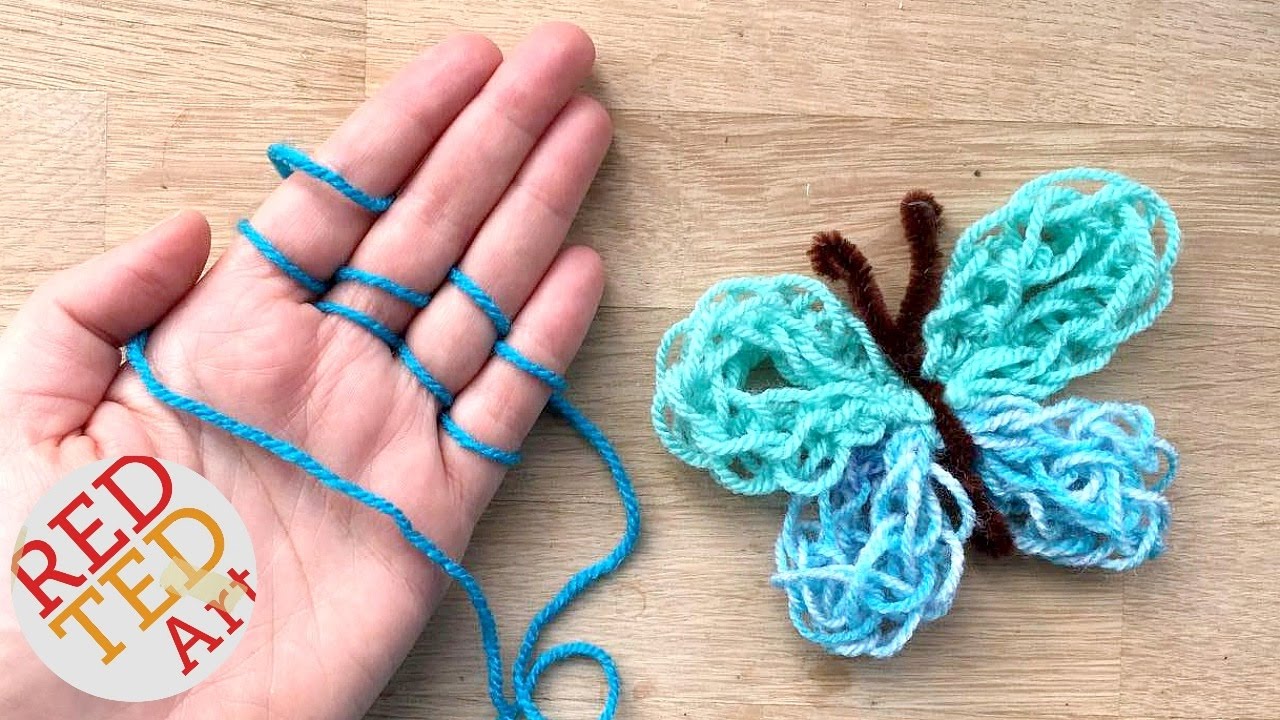This is a detailed photograph featuring a creatively crafted yarn butterfly and a person's hand. The hand, belonging to a white person, is positioned with the palm facing up and interwoven with blue yarn between the fingers. This hand extends from the lower left-hand corner and is placed on a light brown wooden surface that resembles planked flooring.

Next to the hand on the wooden surface is an artfully made butterfly, constructed from various shades of light blue and whitish yarn. The butterfly has two upper wings made from light blue yarn and two slightly darker lower wings. The center body and antennae of the butterfly are fashioned from twisted black pipe cleaners.

In the lower left-hand corner of the image is a white circular logo at a 45-degree upward angle. This logo reads “RED TED ART,” with "RED" in all-red uppercase letters, "TED" in orangish-brown uppercase letters, and "ART" capitalized but not in all caps, also in red. This artistic setup highlights both the intricate yarn work and the branding of the creative project.